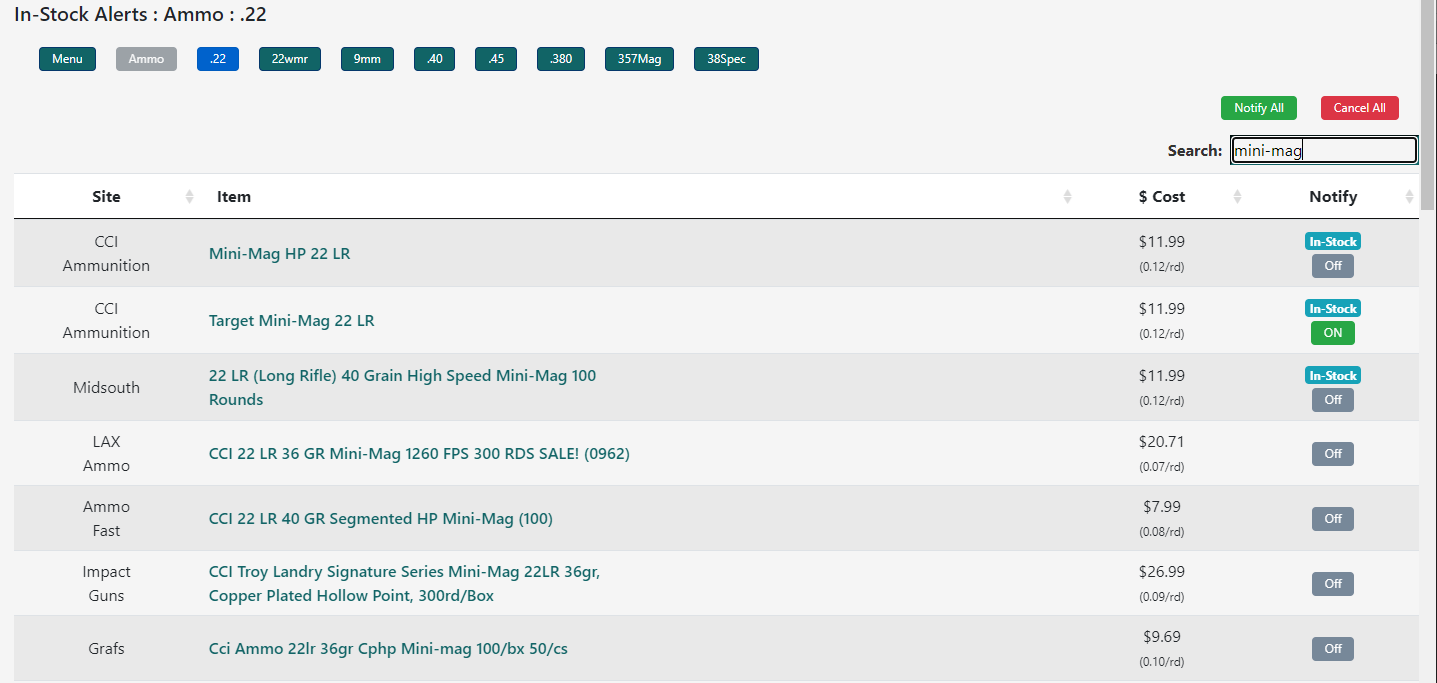This image showcases a detailed screenshot of a website with a primary focus on managing ammunition alerts. The layout is in landscape orientation, approximately twice as wide as it is tall. The background is predominantly gray, with a vertical gray scroll bar on the right side of the page.

At the top of the webpage, in bold black font, it reads "In Stock Alerts Ammo .22." Below this heading, there are multiple clickable boxes for selecting different types of ammunition. The first box is green with white text, followed by a grayed-out ammo box with white text. Additional clickable boxes are color-coded and labeled, including a blue box labeled ".22", a box for ".22 WMR," and other boxes for "9mm," ".40," ".45," ".300," ".357 Mag," and ".38 Special." These boxes likely serve as filters for sorting the ammunition options.

To the right of these filter boxes, there are two prominent buttons: a green box with white text that says "Notify All" and a red box with white text that says "Cancel All." Below these buttons, there's a search bar with a white background and a black border, containing the text "Mini Bag."

Further down, the webpage is organized into several columns with specific headers: "Site," "Items," "Dollar Cost," and "Notify." Under the "Site" column, gray text lists the websites offering the ammunition. The "Items" column features blue text specifying the types of ammunition available. The "Cost" column indicates the price in dollars, and the "Notify" column provides links for users to subscribe to stock alerts.

Overall, the webpage is designed to help users efficiently monitor and select various types of ammunition, with clear options for notification and management.